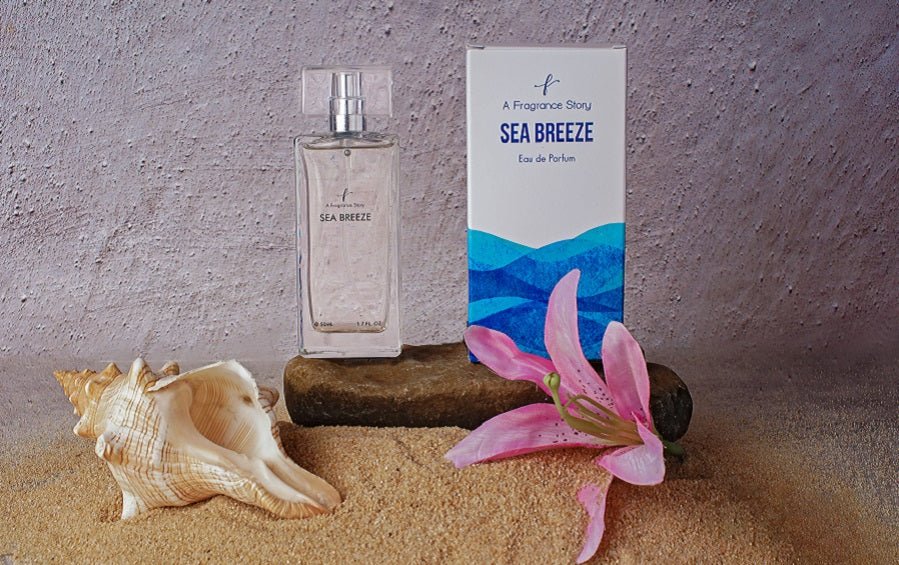This photograph showcases a fragrance advertisement for "Sea Breeze" in a striking beach-themed setting. The perfume bottle, which is a tall, rectangular spray bottle, features a glass bottom and a square plastic top, prominently displaying the text "Sea Breeze" along with the smaller print "a fragrance story" above it. Beside the bottle is the packaging box, which is white with a blue water ripple design and adorned with French words. The box also features the text "a fragrance story" in blue, as well as "Sea Breeze" in larger blue letters and "You Do Perfume" below it. The display elements include fine brown sand, a rock, a white and gold conch shell, and a pink flower situated under the box. The scene is set against a backdrop of a white wall with subtle black marks, effectively highlighting the fresh, coastal theme of the fragrance.